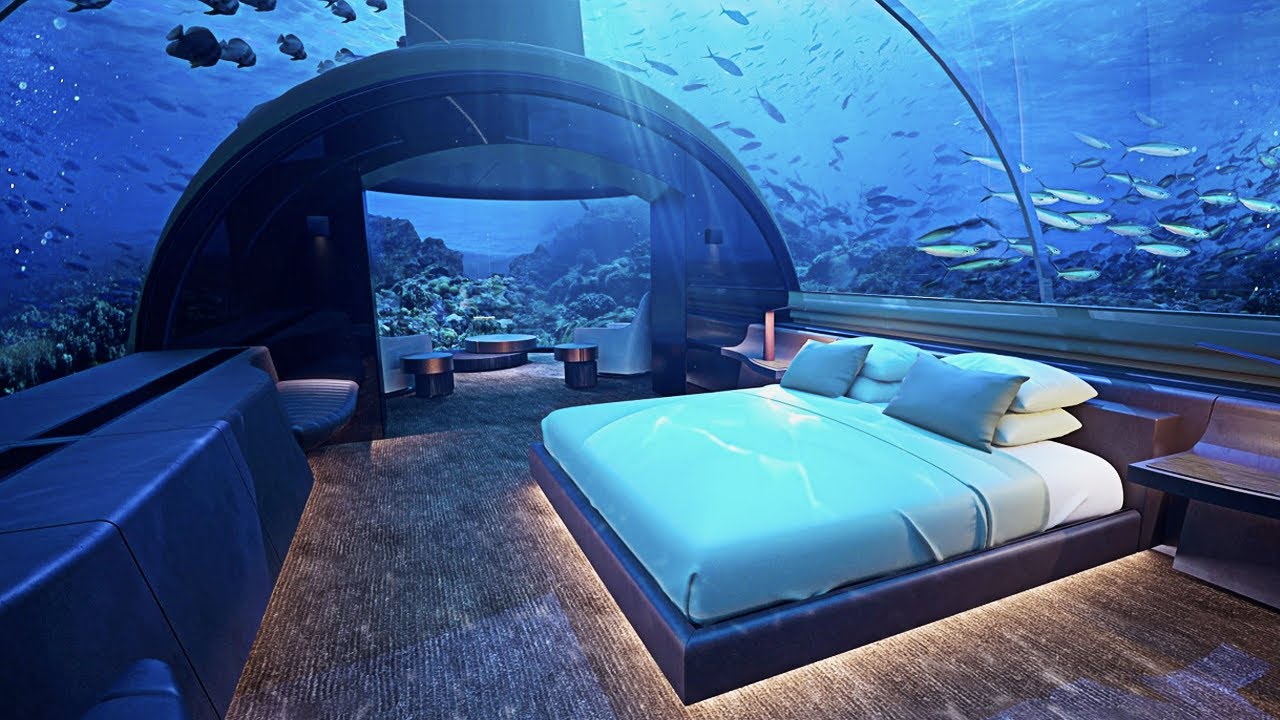The image depicts an elaborate underwater bedroom encapsulated within a transparent, dome-shaped structure. Through the clear walls and ceiling, one can see an array of fish swimming gracefully in the surrounding blue water, illuminated by sunlight filtering down from the surface. The room itself features a wide bed positioned against the right wall, adorned with four white pillows and two gray ones. Beyond the bed, a hallway leads to what appears to be a kitchen or living room area, furnished with white chairs and a distinctive copper, circle-shaped table. The floor of the bedroom seems to be made of grooved steel, lending an industrial touch to the sleek, modern aesthetic. Vegetation and coral reefs can be seen outside the glass dome, adding to the surreal, aquatic ambiance of the space. The image, which might be computer-generated, portrays a mesmerizing blend of design and nature in an underwater habitat.